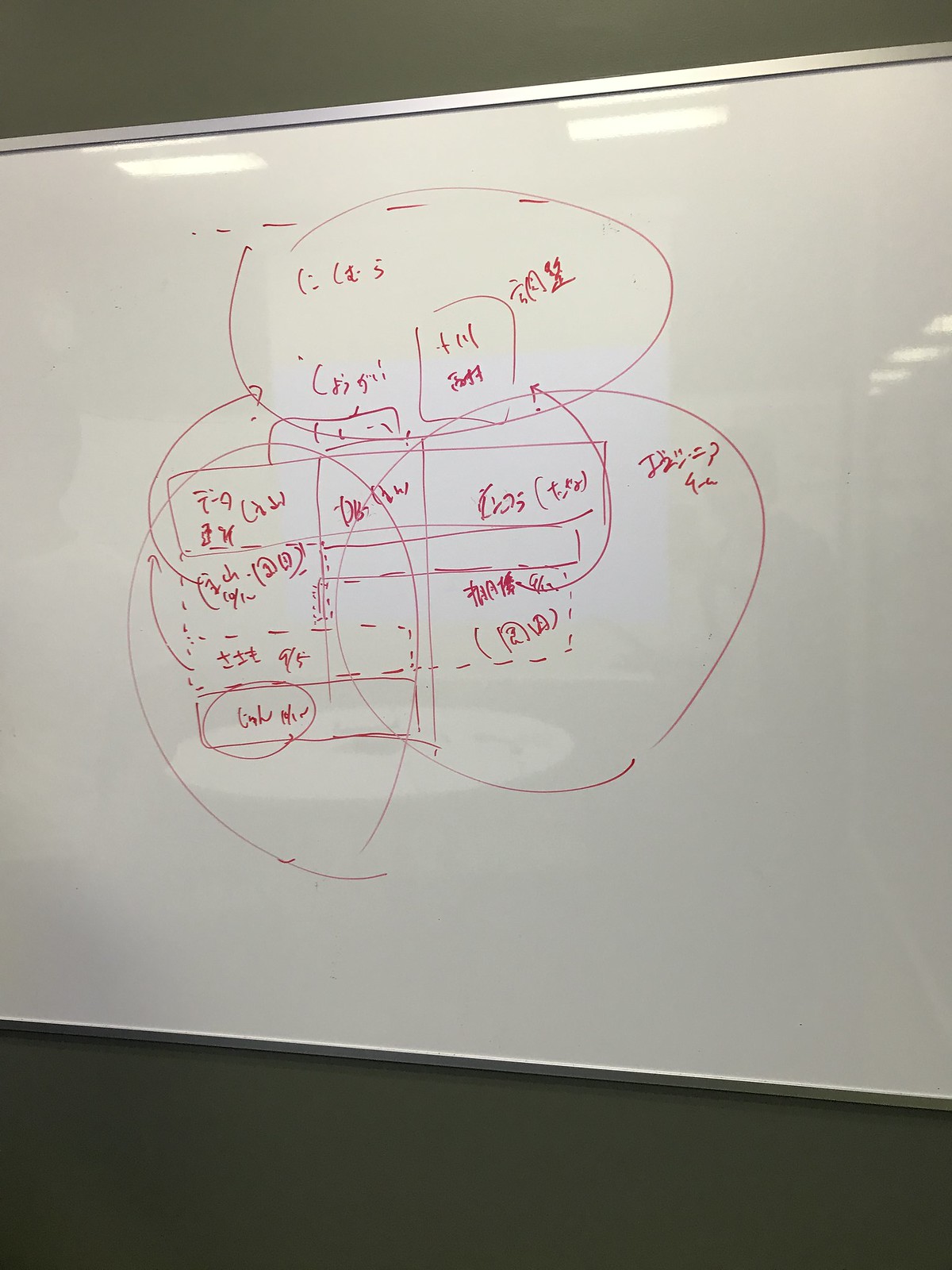The photograph depicts a well-used whiteboard, likely situated within a classroom setting, with red dry erase marker designs and text written across its surface. The whiteboard features a series of geometrically precise shapes, including several rectangles, circles, and directional arrows. Three prominent circles are present, seemingly dividing or categorizing different elements of the illustration. The accompanying text, written in Japanese, remains untranslated. Overhead light sources illuminate the scene, their reflections visibly cast onto the whiteboard. Though there are no people directly in view, faint reflections of individuals and a centrally positioned table within the classroom can be discerned.